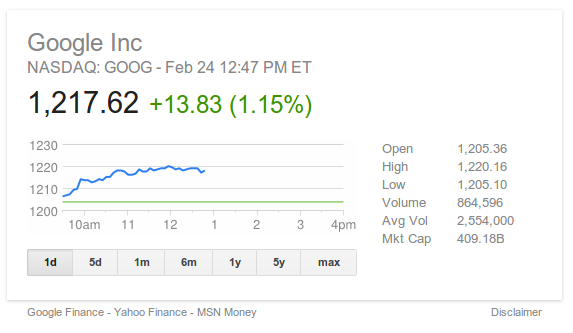A detailed screenshot from Google Finance displays the stock information for Google Inc. At the top, "Google Inc." is written in gray letters, followed by "NASDAQ: GOOG - Feb 24, 12:47 p.m. ET" in slightly smaller text. Below that, in black, the stock price is prominently displayed as "1217.62," accompanied by a smaller green text showing an increase of "+13.83 (+1.15%)."

The center of the screenshot features a small graph charting the stock's performance throughout the day. The graph includes a blue line that trends upward incrementally, though it is jagged with fluctuations. Below the blue line, a steady green line hovers within the range of $1200 to $1210. On the x-axis, time is marked from 10 a.m. to 4 p.m., while the y-axis spans from $1200 at the bottom to $1230 at the top, with markers at $1210 and $1220.

On the far right, smaller gray text outlines the stock's key metrics in the following format: 
- Open: 1205
- High: 1220
- Low: [value not specified]
- Volume: [value not specified]
- Avg Volume: [value not specified]
- Market Cap: [value not specified]

At the bottom of the screenshot, various selectable time frames are listed, including "1D," "5D," "1M," "6M," "1Y," "5Y," and "Max," with "1D" currently selected. Finally, in gray letters at the bottom, the sources are cited as "Google Finance - Yahoo Finance - MSN Money."